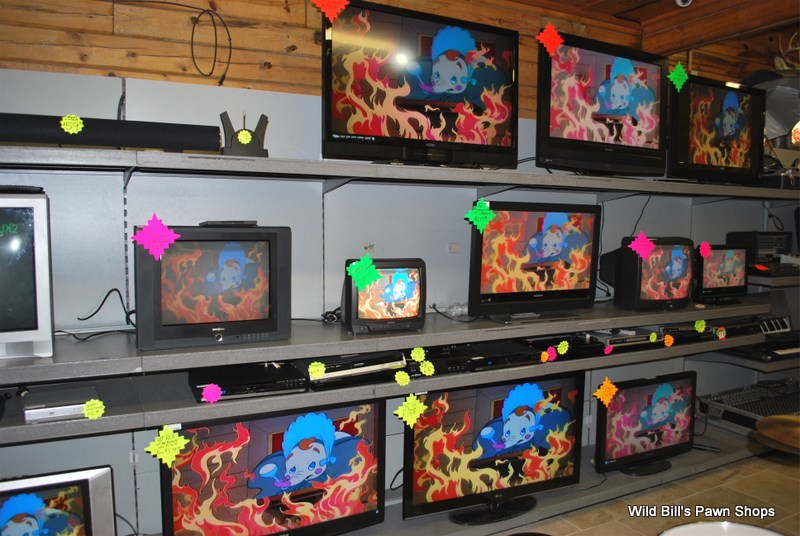The image depicts the interior of Wild Bill's Pawn Shops, a store specializing in second-hand electronics. The store is dimly lit, with light yellowish-brown tiled flooring and visible wooden beams on the ceiling. The white walls and silver metallic shelving units hold an array of televisions in various shapes and sizes. Some of the TVs are flat-screen models with either black or silver bezels, while others are older tube models.

All televisions display the same cartoon scene, featuring a crying baby elephant in a flaming room, likely a scene from the movie 'Dumbo'. Each TV bears a brightly colored, diamond-shaped sticker on the top left corner—colors include neon pink, green, yellow, orange, and red—none of which display visible prices.

In addition to the televisions, flat rectangular electronics, possibly DVD players or CD players, are situated on one of the shelves between the two bottom levels of TVs. The bottom shelf also contains what seems to be a soundboard for studio equipment. The words "Wild Bill's Pawn Shops" are emblazoned in white text at the bottom right-hand corner of the image, confirming the nature and ownership of the establishment.